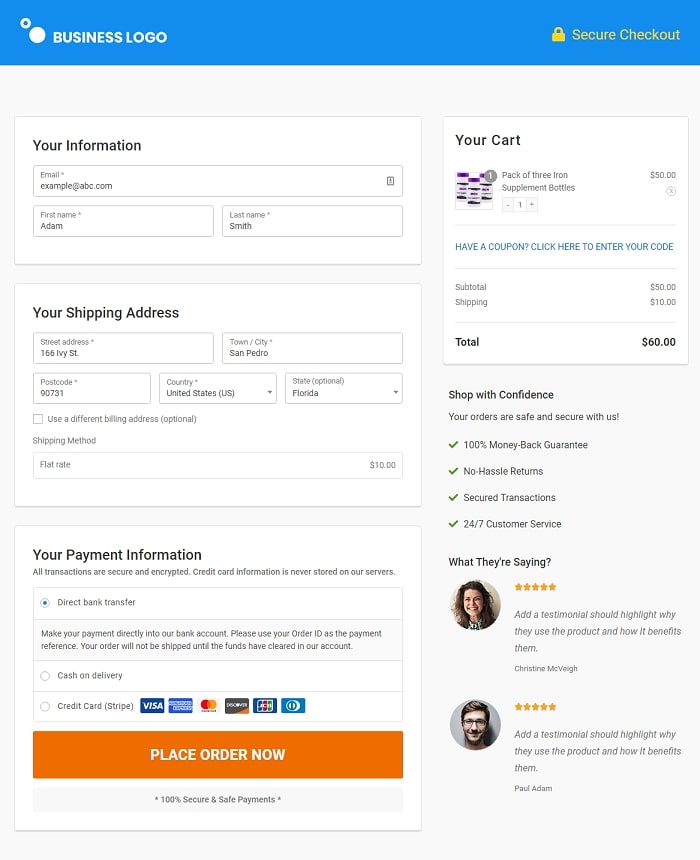**Detailed Descriptive Caption:**

The image captures a screenshot from a website featuring an online checkout page. At the top, there's a medium blue banner containing two circles; one is an outlined circle with a hole in the middle, and the other is a solid circle. Adjacent to these circles is the text "BUSINESS LOGO" in all capital letters. Moving to the right of the banner, there's a yellow padlock icon accompanied by the text "Secure Checkout" in yellow print, with both words capitalized.

Below the banner, the page background transitions to light gray, with various white rectangular sections dividing the content. The first section, titled "Your Information," prompts the user to input their email address, first name, and last name. Beneath this is the "Your Shipping Address" section, which requests details such as street address, town/city, postcode, country, and state. A checkbox option labeled "Use a different billing address" is available as well, marked optional in parentheses.

Following this, the "Shipping Method" section indicates a flat rate shipping fee of $10. The next section, "Your Payment Information," provides several payment options: credit card, cash on delivery, and direct bank transfer. At the bottom, an orange banner with white text invites the user to "Place Order Now."

On the right side of the checkout page, the "Your Cart" summary displays a pack of three iron supplement bottles priced at $50. A prompt for entering a coupon code is included, along with a detailed cost breakdown: a subtotal of $50, a shipping fee of $10, bringing the total to $60.

Additional assurances highlight the shopping experience with statements such as "Shop with Confidence," "No Hassle Returns," "100% Money Back Guarantee," "Secure Transaction," and "24/7 Customer Service." The page also features customer feedback, showcasing two reviews under the "What People Are Saying" section.